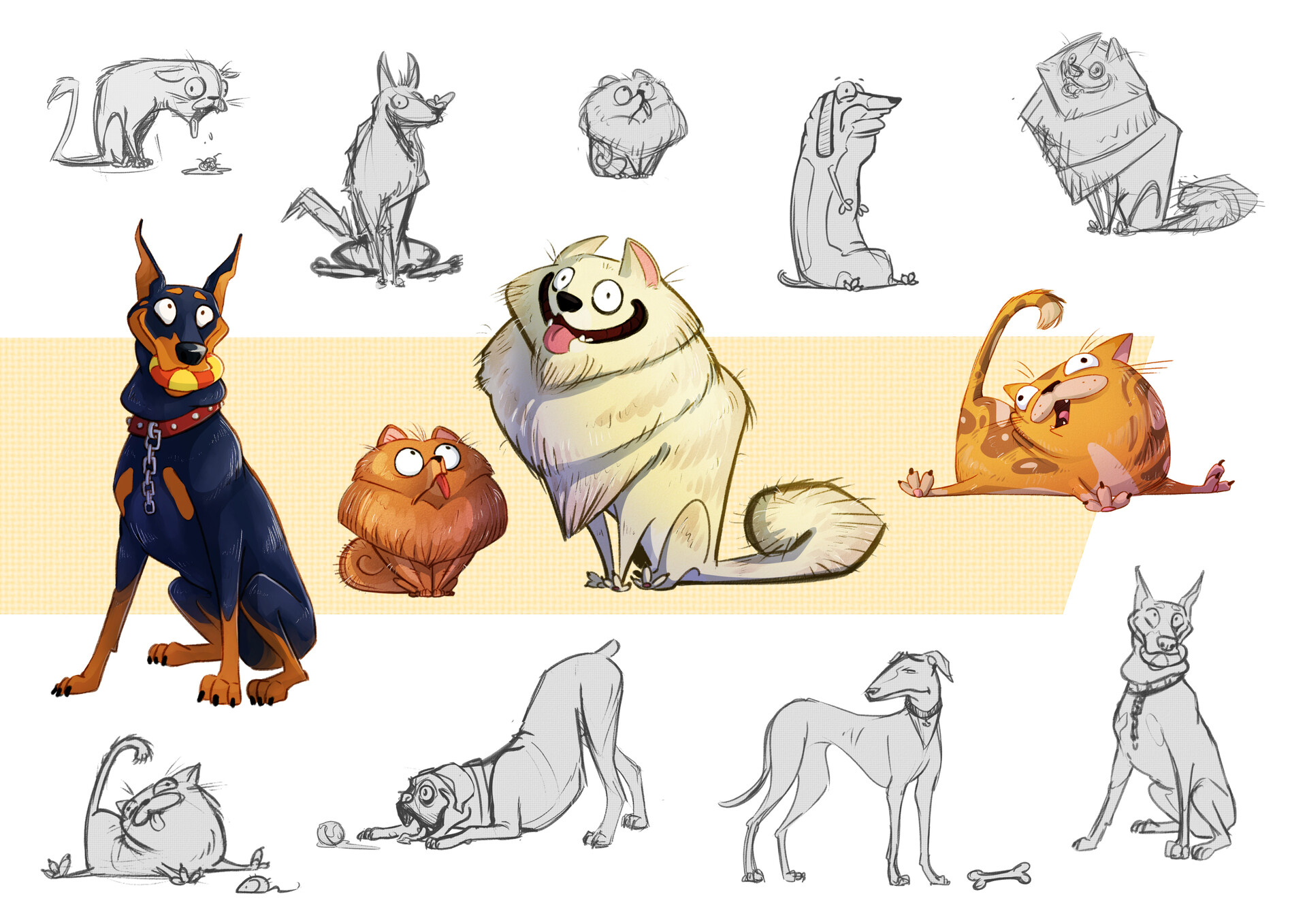The image showcases a series of cartoon-like drawings of various animals, predominantly dogs and cats, arranged in three rows. The top row consists of five hastily sketched, black and grey illustrations. From left to right, it features a cat vomiting a hairball, a happy medium-sized dog, a small toy-like dog with its tongue sticking out, a distressed beagle sitting on its rear end, and a smiling husky.

The middle row, which is in color and appears to be the focal point, starts with a black and brown Doberman Pinscher wearing a red collar and chain. The Doberman is holding a yellow and red toy in its mouth. Next to it is a small, fluffy Pomeranian-looking dog staring up adorably. In the center is a large, happy white dog with pink ears, a big black mouth, and a pink tongue. To its right is an orange cat lying on its belly with its front paws stretched out in front and back paws splayed out, looking mildly distressed with its tail raised and crooked.

The bottom row consists of more sketch-like black and grey drawings. It depicts a repeat of the orange cat with a toy mouse in front of it, a playful dog in a typical play pose with a ball, a snooty-looking greyhound glancing away with a bone in front of it, and a preliminary sketch of the Doberman from the middle row, drawn in the same style but without colors. Centered in the middle of the image is a yellow bar. Overall, the collection is a blend of whimsical, cartoonish representations of animals, totaling thirteen characters in varying expressions and poses, clearly emphasizing the animated, clip art style.